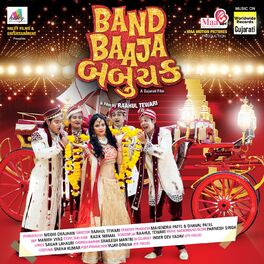The image depicts the cover of an Indian music album titled "Band Baaja Giririf" ('Band Baja Chorus' is also noted but less consistent across the descriptions). The cover features a vibrant and colorful scene with a predominantly red background, including a red staircase and an antique red car. Centered prominently in the image are five individuals, dressed in traditional and vibrant attire. The group consists of one woman and four men. The woman, positioned front and center, is adorned in a cream-colored dress with a red shawl and has dark black hair, adding to the traditional Indian aesthetic. Surrounding her, the men stand in white jackets with black pants, and two of them are accessorized with yellow leis. The image is detailed with orange letters in a script resembling Arabic, spelling out the album's title on a brightly designed backdrop. The corners of the cover feature various colors and symbols, possibly indicating sponsorships or creators of the album, with additional text in what could be Gujarati.